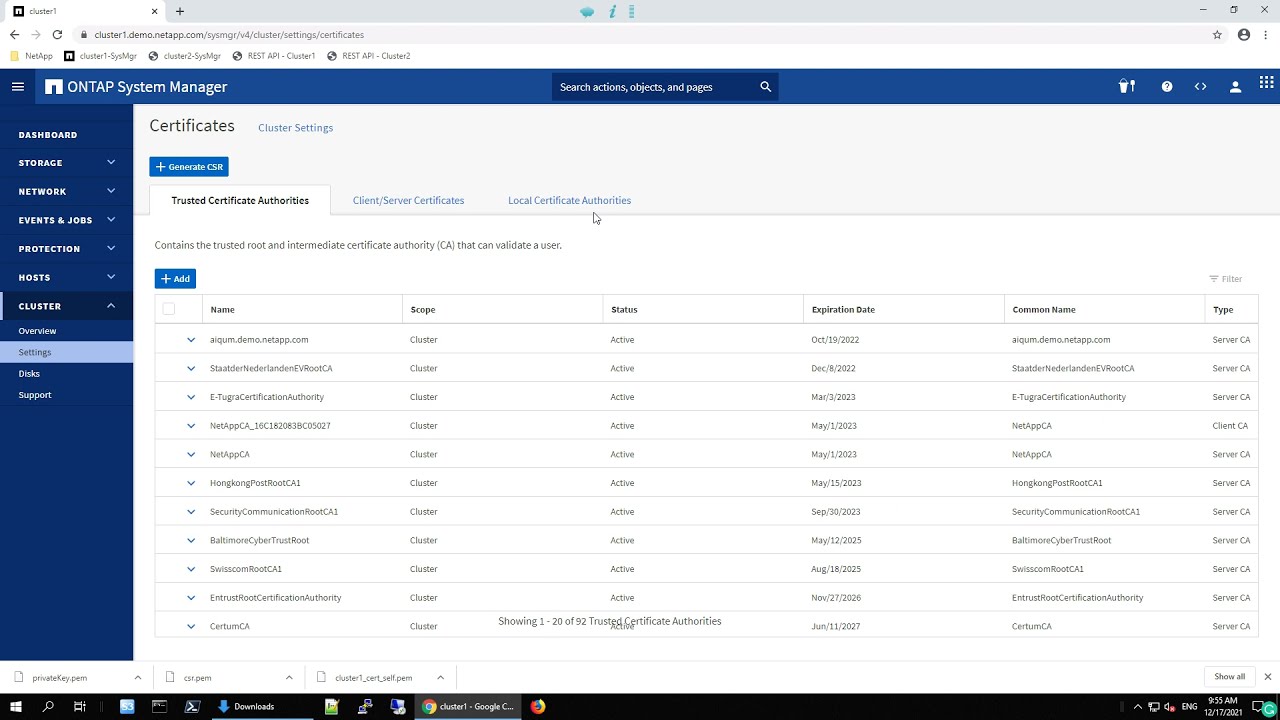The image captures the screen of a Windows computer with the Google Chrome browser open, displaying a system manager web application. The webpage features distinctive blue borders on the left and right sides, and a search bar is positioned at the upper left corner. "ONTAP System Manager" is prominently displayed in white text against a black, red, and blue background at the top of the webpage. Along the left side, in a vertical white menu against a blue background, are several navigation items including Dashboard, Storage, Network, Events and Jobs, Protection, Hosts, Cluster Overview, Settings, and Disk Support.

In the main white-centered area with black print, the heading "Certificates" is located in the upper left corner. Below it, various menu options are listed, such as "Generate CSR," "Trusted Certificate Authorities," "Client Server Certificates," and "Local Certificate Authorities," with additional descriptive text explaining their function, and an "Add" button.

The content includes a table displaying columns titled Name, Scope, Status, Expiration Date, Common Name, and Type. Examples of entries under these columns are certificates with names like "AIQM.demo.netapp.com" and "STAAT DER NEDER LANDEN EV Root CA," all with a scope marked as "Cluster" and statuses marked as "Active." The expiration dates range from 2002 to 2027, and types include "Server CA," "Service CA," and "Client CA." The table indicates that it is showing 1 of 20 of 92 trusted certificate authorities.

The bottom of the screen shows the taskbar with familiar Windows icons, such as the Windows symbol, search icon, and the Google Chrome icon. Additionally, it displays the time and date, "12:17 12/17/2021," near the bottom right corner. The taskbar and browser elements like the downloads icon and navigation tools in the bottom portion support the setting of this being a typical computer screen view while accessing a system manager tool.